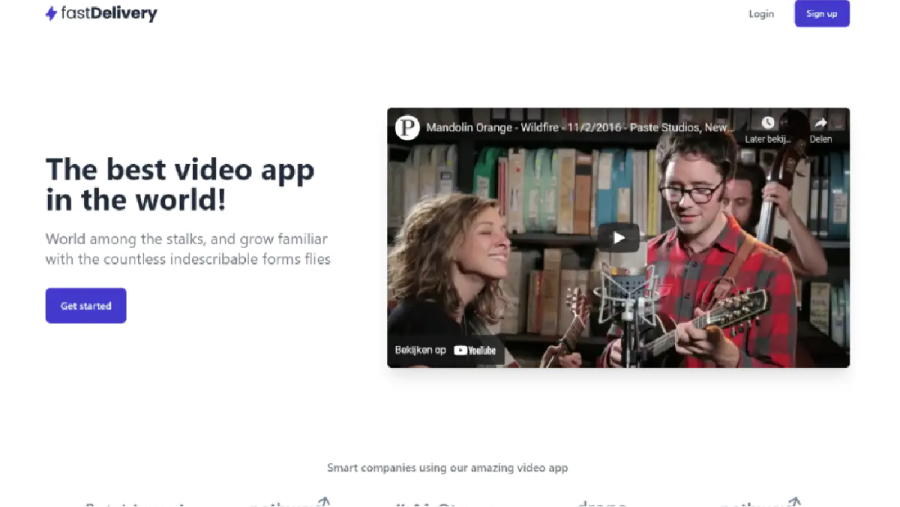This computer screen capture, taken from a webpage, prominently features the phrase "Fast Delivery" at the top. In the upper right corner, there is a login section and a blue "Sign Up" button. Moving down to the center of the page, on the left side, it reads: "The Best Video App in the World. World among the stocks, world among the stocks, and grow familiar with the countless indescribable forms, flies." Below this text is a blue "Get Started" button. 

On the right side of the page, there is an embedded YouTube video. The thumbnail shows a man playing a guitar alongside a woman, with another man in the background. The video title is "Mandolin Orange - Wildfire," dated "11/2/2016," and labeled "Paste Studios, New." The thumbnail also features a play button.

At the bottom of the screen, though partially cut off, there is a visible section stating, "Smart companies using our amazing video app." The following lines are not fully visible, leaving the text incomplete.